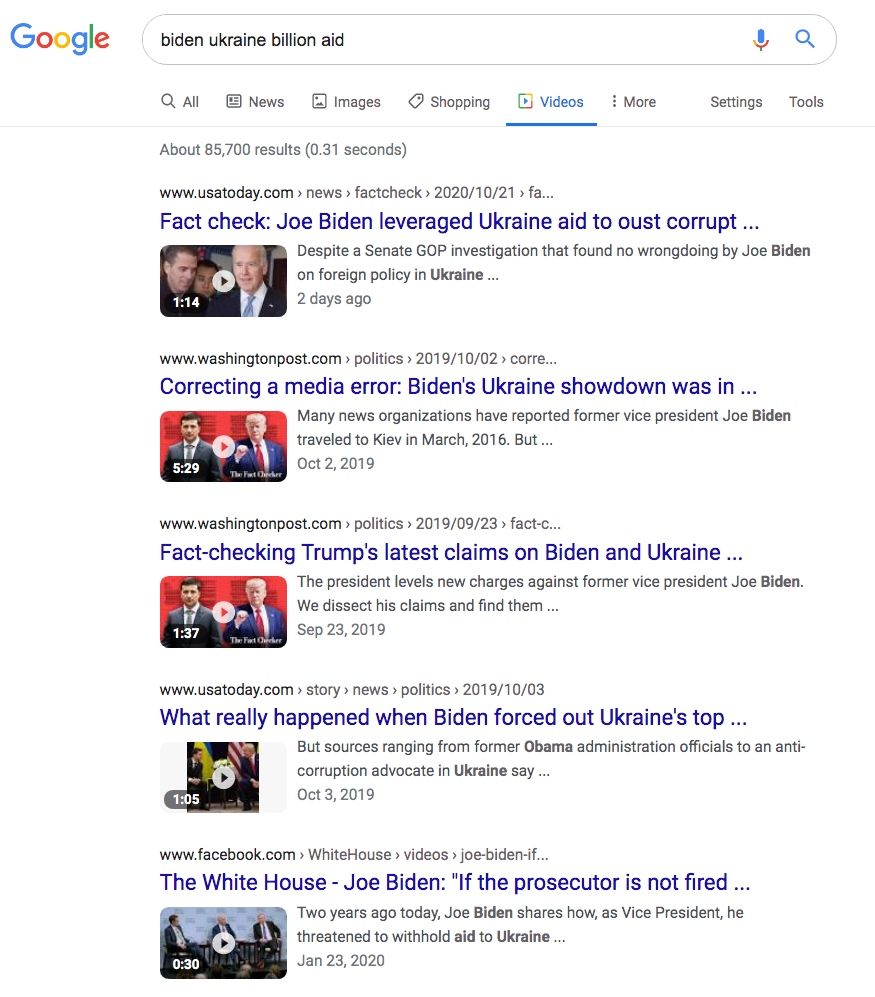The image is a screenshot of a Google search results page. In the upper-left corner, the signature Google logo is prominently displayed. Immediately to the right of the logo is the search bar, within which the query "Biden Ukraine Billion Aid" has been entered. Below the search bar, the search results are displayed, specifically tailored by the selection of the video tab for the query.

The top five video search results for "Biden Ukraine Billion Aid" are shown. The first result is from USA Today, followed by the second and third results from the Washington Post. The fourth result is again from USA Today, while the fifth result is from Facebook. Each search result is accompanied by preview thumbnails indicating they are video content. Notably, the total number of results returned for this query is approximately 85,700.

The layout is typical of a Google search results page, with the emphasis on video content clearly visible due to the selected filter. The screenshot captures a snapshot of the immediate and diverse media response to the query related to Biden's aid to Ukraine.